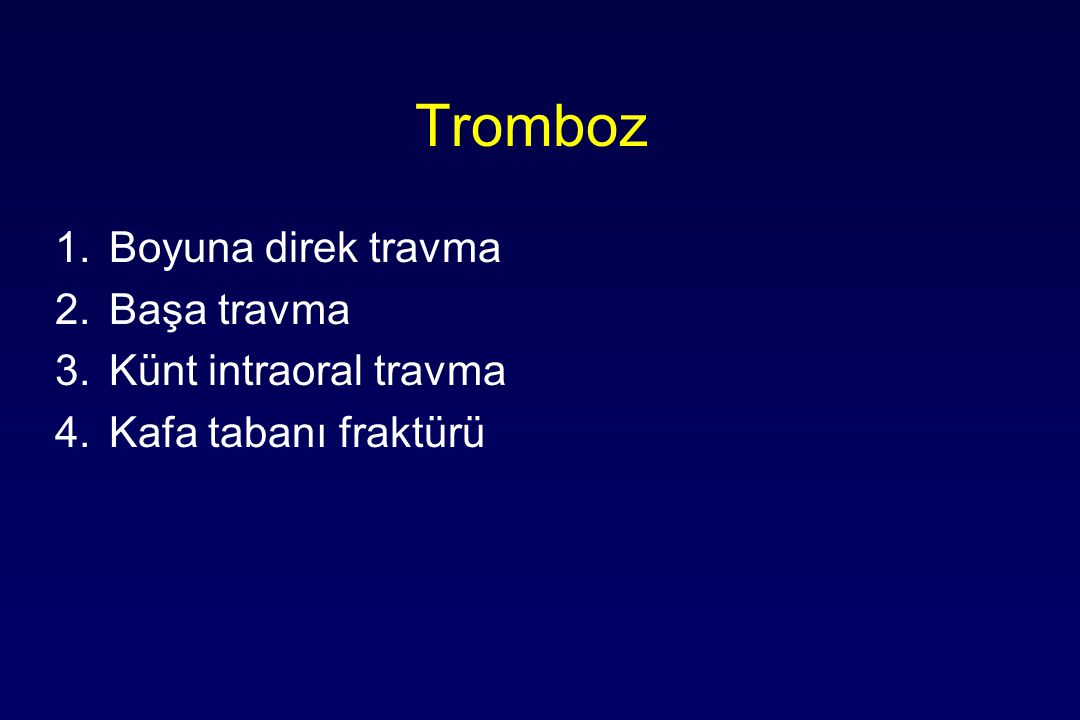The image is a horizontal rectangular slide from a PowerPoint presentation, featuring a dark blue to bluish-purple gradient background. At the top center of the slide, a yellow title reads "TROMBOZ" in a slightly larger and skinny font, spelling out T-R-O-M-B-O-Z. Below this heading, there are four points listed in white text, aligned neatly to the left. Each point is numbered from 1 to 4 and is written in a foreign language. The text for these points is slightly smaller and thinner than the title, with each point beginning with a capital letter and consisting of 2 to 3 words per line. The points do not have periods at the end of each sentence, and the content of these points is unclear due to the unfamiliar language. The textual content occupies the top third of the image, while the rest of the slide remains the darker blue background.